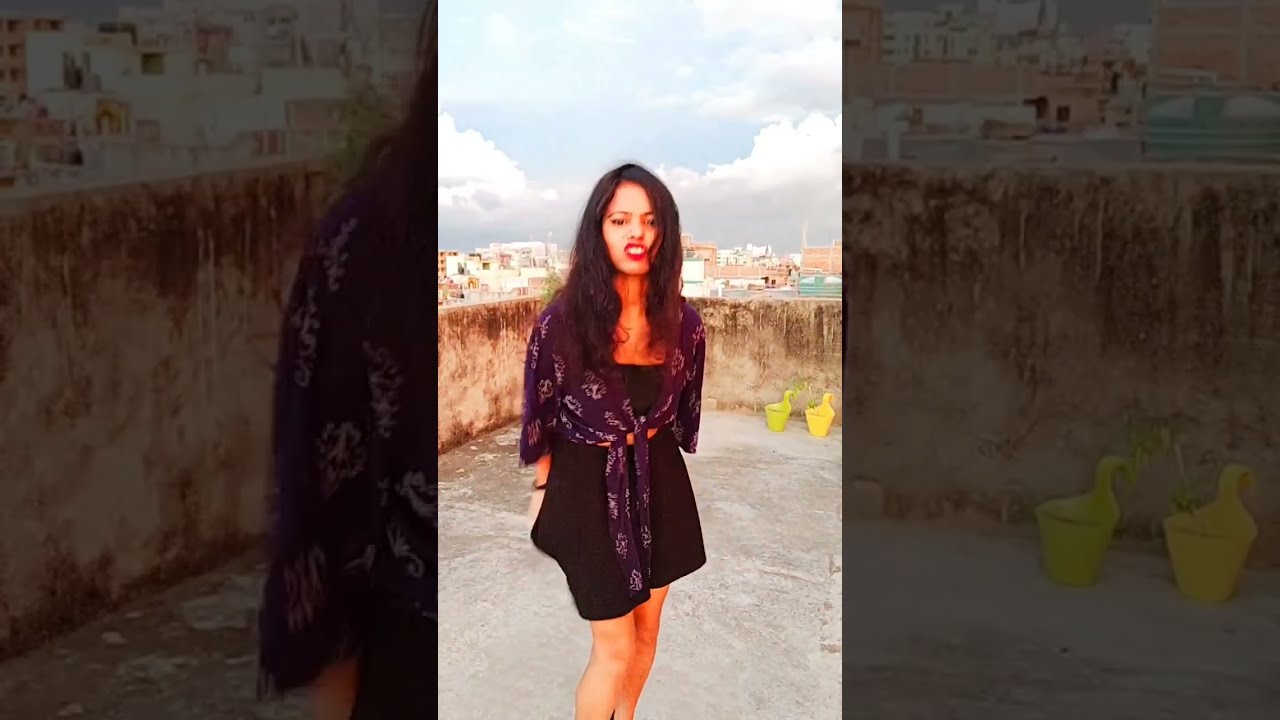The photograph features a woman standing on a worn, aged concrete rooftop against a faded cement wall. She is dressed in a black mini dress paired with a purple shawl draped over her shoulders. Her long brown hair frames her face which sports bright red lipstick, and she is making a kissy face at the camera. The background shows a partly cloudy day with patches of a blue sky, and a distant city skyline of white buildings with no skyscrapers. On the right side of the image, two yellow buckets with bent handles are positioned against the wall. The photo has been edited to create a darkened, enlarged frame on both the left and right sides, resulting in a split view where only parts of the woman and the rooftop context are visible.